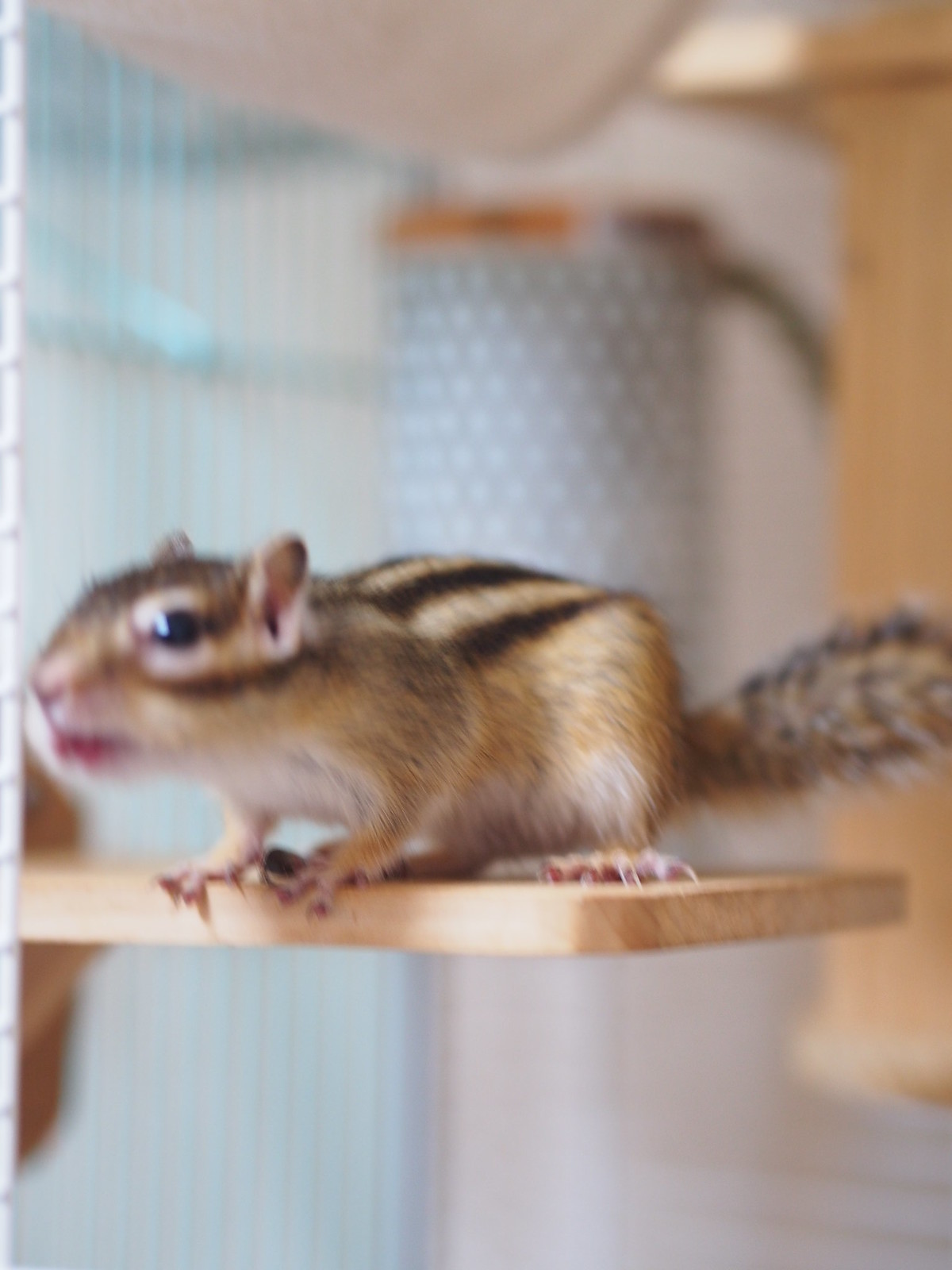This image features a chipmunk indoors, possibly in someone's house or in a store, perched on a brown pine shelf that's attached to a glass or plastic wall. The chipmunk appears to be holding a black seed in its left front paw. Although the overall image is blurry, the chipmunk is front and center with its body facing forward and its nose close to the right edge of the photo. The animal's bushy tail extends off the back of the shelf towards the left. Its fur is tawny and white with dark brown stripes along its back, complementing its black beady eyes and small ears. The background is indistinct, showing vague shades of blue and some undefined wooden and round structures, adding to the indoor setting ambiance.